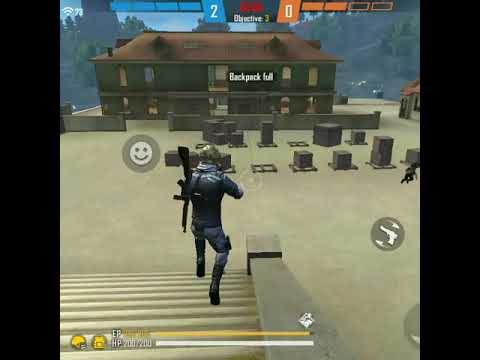The image is a screenshot from a video game featuring a horizontally rectangular screen with black bars on its left and right edges. The main scene shows a character in military gear, wearing dark blue and gray clothes, black boots, a helmet, and a rifle slung over his left shoulder. He is captured mid-action, jumping or running down a set of stone stairs toward a gray plaza filled with various cubic and rectangular gray structures.

The background features a large rectangular army green building with a brown or reddish triangular roof, set against a backdrop of tree-covered mountains. Over this building, white text reads "backpack full." 

The top of the screen displays a scoreboard with two blue bars on the left showing the number two, and two orange bars on the right showing zero, with the text "objective three" in the middle. At the bottom of the screen, a series of energy or life gauges in yellow and white are nearly full, accompanied by white text indicating hit points at "200/200." Additionally, there are some yellow icons in the bottom left corner.